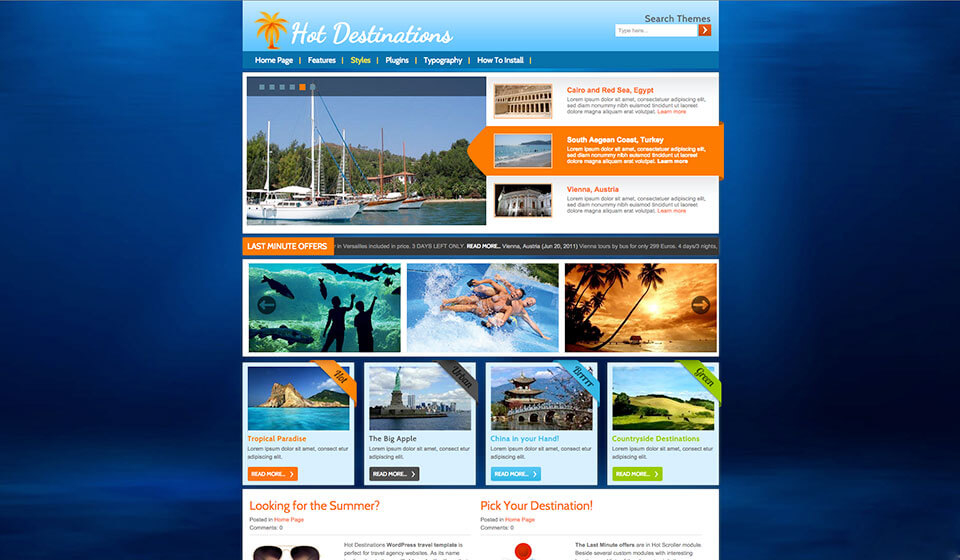The caption has been transformed into a detailed and organized description:

---

The image depicts a travel destination website that caters to individuals and families seeking vacation spots. The header features an eye-catching orange and red palm tree with the text "Hot Destinations." To the right, there is a search bar for exploring themes. Below the header, navigation options include Home Page, Features, Styles, Plugins, Topography, and Installation Guide.

Currently, the focus is on "Styles." A vivid image displays sailboats docked at a marina, representative of South Asian coastal areas in Turkey, although the text beneath is in an unreadable language. The section also highlights various international destinations, such as the Cairo Red Sea in Egypt and Vienna in Austria, each with a "Learn More" button.

Further down, an orange button labeled "Last Minute Offer" is prominently displayed. Adjacent to this are images showcasing various activities: people observing marine life in an aquarium, a family enjoying a water slide, and a picturesque sunset framed by palm trees. 

The subsequent section presents a variety of destination types. A "Tropical Paradise" option encourages further exploration, labeled as a "Big-Ticket Item." An "Urban Experience" showcases a bustling cityscape, and a "Green Travel" option highlights eco-friendly vacation spots.

At the bottom of the image, additional information about choosing destinations and planning summer vacations is provided. The section includes details on who posted the content, offering guidance and insights for travelers.

---